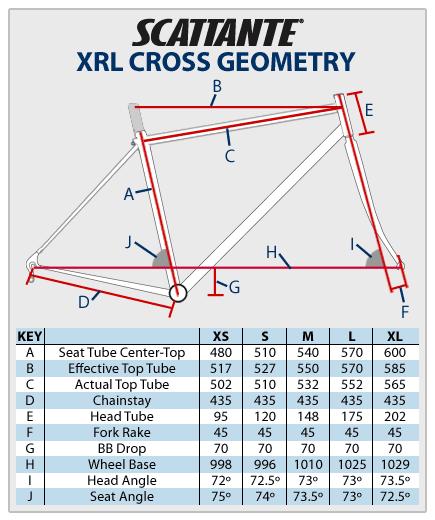This is a tall rectangular image featuring a detailed schematic and chart for a cross-country bike made by Scatante. The background is light gray with a thin darker gray border encasing the entire graph. At the top, in italicized all capital letters in black font, it reads "SCATANTE," and directly below, in bold blue capital letters, it reads "XRL CROSS GEOMETRY." The diagram beneath these titles displays a schematic of the bike, marked with several lines in white, red, and gray, labeled with letters from A to J. Each labeled point corresponds to specific parts and measurements of the bike's geometry.

The diagram provides detailed annotations indicating various points on the bike: 
- "A" for the seat tube center top
- "B" for the effective top tube
- "C" for the actual top tube
- "D" for the chainstay
- "E" for the head tube
- "F" for the fork rake
- "G" for the BB drop
- "H" for the wheelbase
- "I" for the head angle
- "J" for the seat angle

Underneath the schematic, there is a chart with seven columns and at least 11 rows, alternating between light blue and white, filled with black font at the head and within the entries. This chart provides specific sizes (extra small, small, medium, large, extra large) and their corresponding measurements. For instance, the seat tube measurements range from 480mm for extra small to 600mm for extra large, and different angles for the seat angle for each size (75° for extra small, scaling down to 72.5° for extra large). The chart and schematic collectively offer comprehensive data on the bike's construction and the various size specifications for each juncture of the frame.